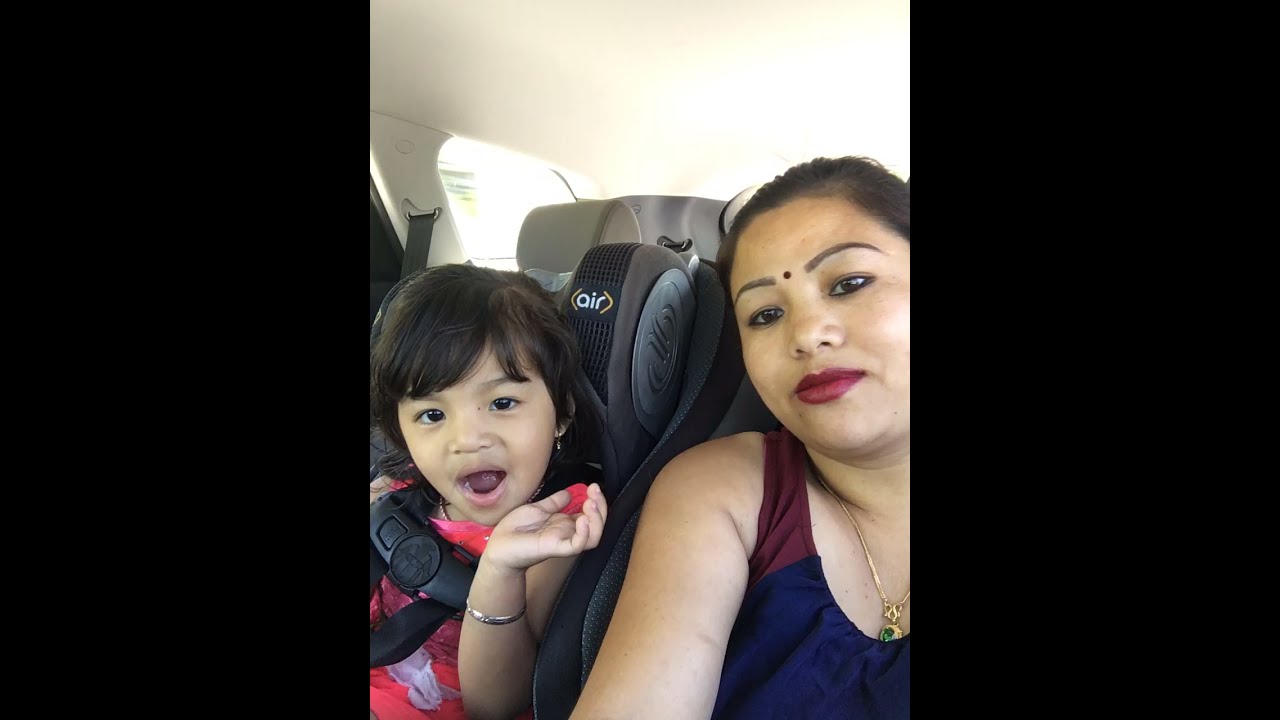In the photo, an Asian woman, possibly of Indian or Pakistani descent, is taking a selfie inside what appears to be an airplane. The woman is wearing a black and purple tank top, sporting red lipstick, and has a red bindi on her forehead. She wears a gold necklace with a green jewel. To her left is a young child, approximately two or three years old, also Asian, dressed in a red and grey striped t-shirt and sporting a bracelet. The child, who might be a girl, is strapped into a child seat and is holding up a hand with an open mouth, possibly reacting to something or holding a toy or candy. The interior of the plane is white, with a window in the background allowing natural light to stream in, giving off a soft, grey lighting. The headrest behind the woman has the word "air" on it, reinforcing that they are indeed on an airplane. It appears that the woman is capturing a moment of their travel.